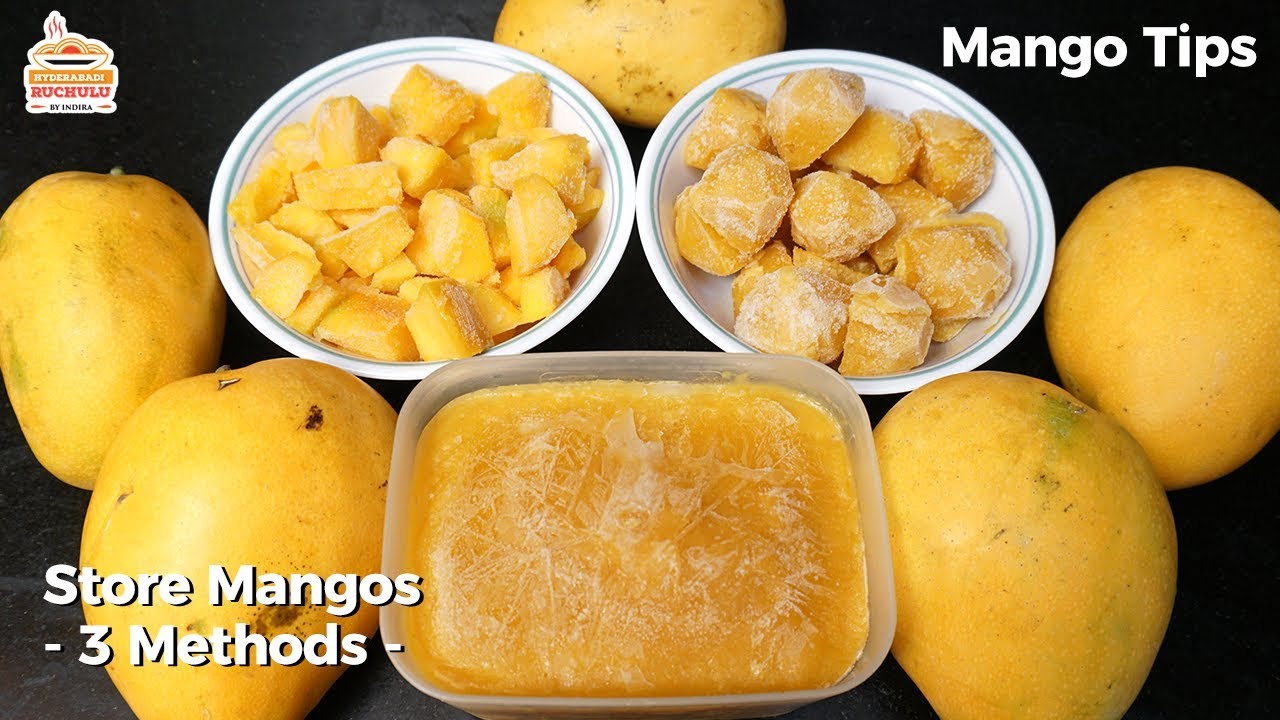The image is a rectangular thumbnail meant for a video titled "Mango Tips." In the top right corner, the text "Mango Tips" is displayed in white letters. The bottom left corner bears the text "Store Mangoes - 3 Methods" in white. The background is black, accentuating the bright yellow and orange hues of the mangoes. The image showcases five whole mangoes arranged on a black surface, with some mangoes slightly cut off at the edges. In the center top, there are two white bowls; the left bowl contains smaller, light yellow mango slices, while the right bowl holds larger, darker yellow dried mango pieces. Below these bowls, a clear plastic container filled with a yellowish solid mass, likely frozen pureed mango, occupies the foreground. At the top left of the image, a logo featuring a bowl with three circular food items and steam rising, bears the text "Hyderabadi Ruchulu by Indira". This thumbnail seems to introduce a tutorial on how to store mangoes using three different methods, presumably set in a kitchen or similar culinary space.